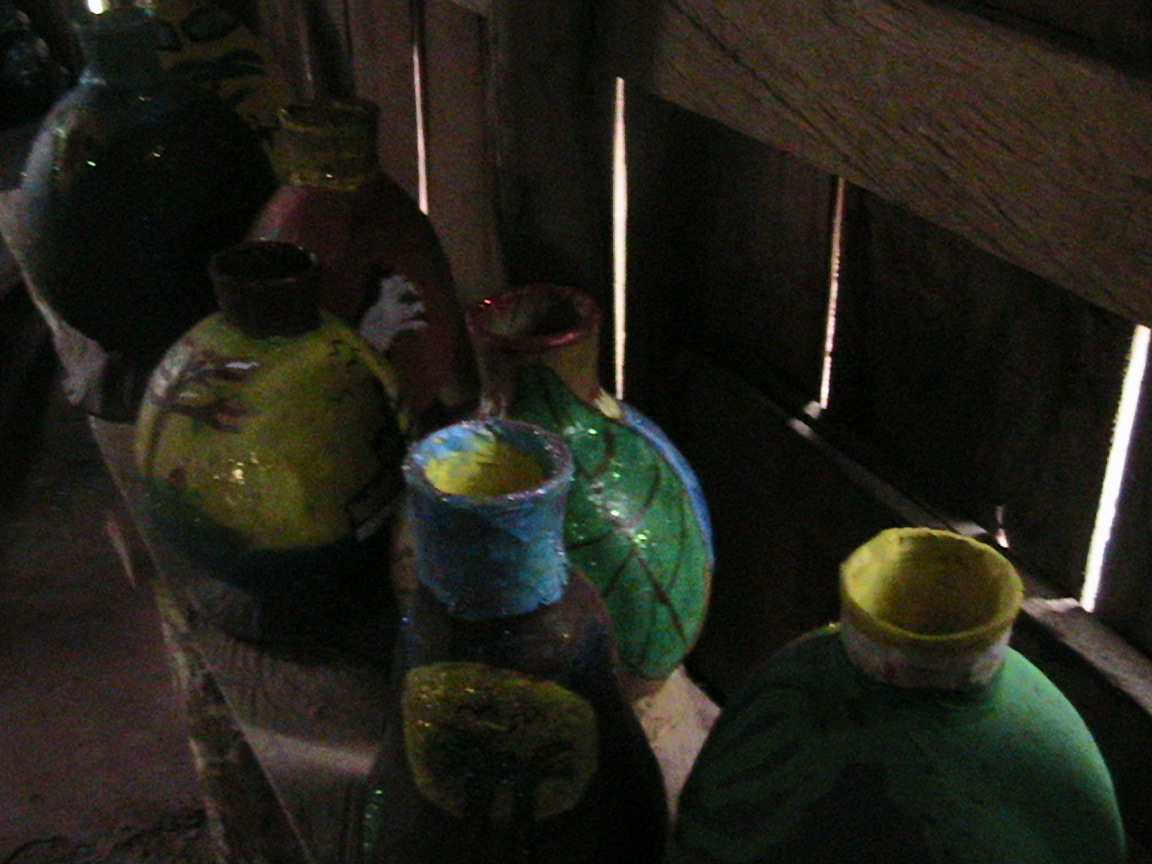This color photograph captures an array of handmade ceramic vases arranged on a dark wooden workbench inside a rustic, dimly lit barn or wooden shed. The wooden walls, made up of wide planks, allow slivers of light to peek through the cracks, casting intermittent beams across the dim interior. The workbench, positioned diagonally from the bottom right corner to the top left, holds a row of six vases, each uniquely painted and roughly a foot tall. 

Starting from the bottom right, there's a large, oval green vase with a yellow cap. Next is a brown vase with a longer blue neck and a yellow circle in its center. Following that, there's a bulbous vase adorned with green, black lines, and blue accents, while a lighter green vase behind it features a brown tree design. Toward the upper left, a red and yellow vase showcases a man's face, partially obscured by another vase. The far left corners house a black and a red vase, the latter with a yellow top. The overall scene is dark, with vases glistening where the light hits them, highlighting their glossy, albeit crudely crafted, surfaces.